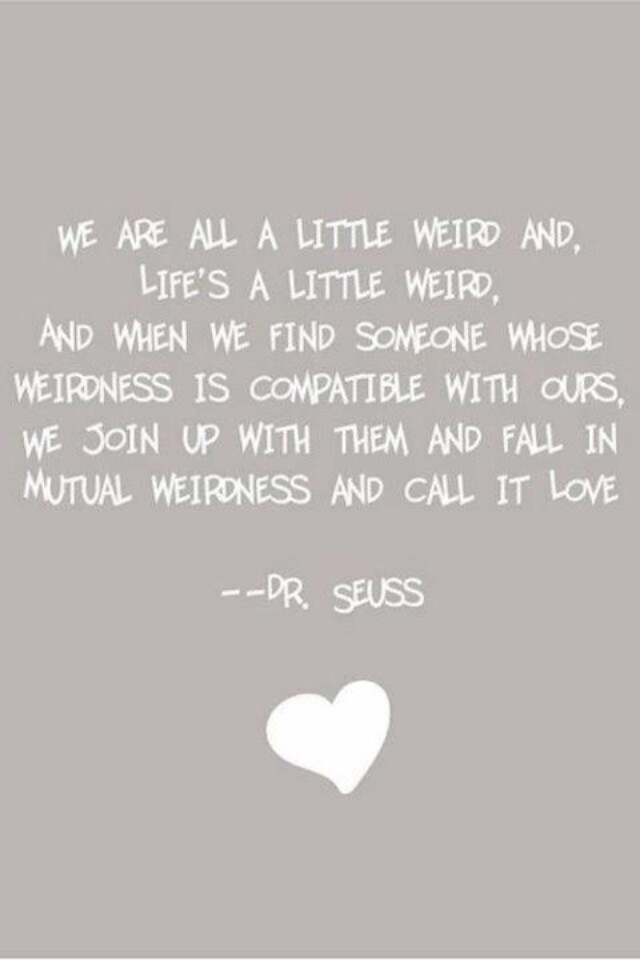The image features a quote attributed to Dr. Seuss displayed on a solid dark gray background. The text is rendered in simple, all capital white letters and begins approximately a quarter of the way down from the top. The quote reads: "WE ARE ALL A LITTLE WEIRD AND LIFE'S A LITTLE WEIRD. AND WHEN WE FIND SOMEONE WHOSE WEIRDNESS IS COMPATIBLE WITH OURS, WE JOIN UP WITH THEM AND FALL INTO MUTUAL WEIRDNESS AND CALL IT LOVE." Below the text, there are two dashes followed by the name "DR. SEUSS." At the very bottom of the image, there is a solid white heart. The overall design gives off a clean, minimalist aesthetic, making it suitable for social media posts, t-shirts, or plaques.